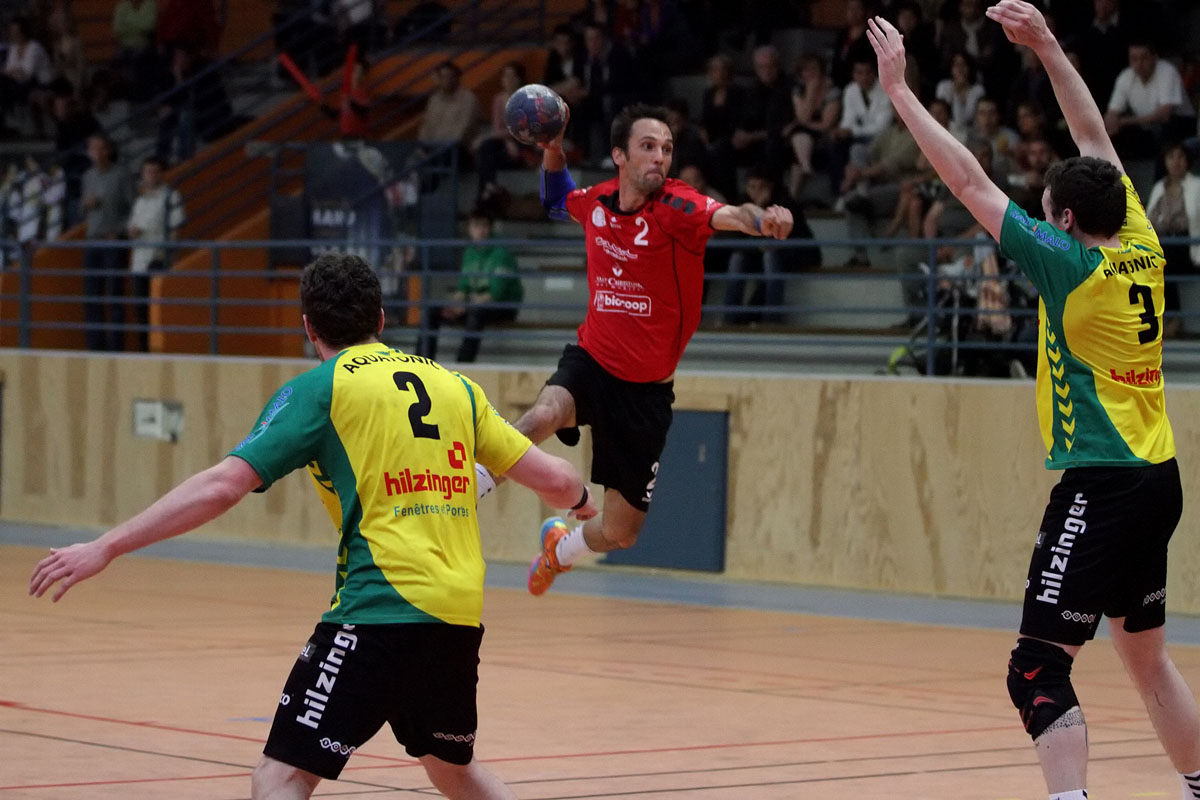In an indoor gymnasium, a dynamic photograph captures a high-intensity moment during a sports game. The action centers on a male athlete in a red shirt with black and white details, paired with black shorts and orange sneakers. He is caught mid-air, clutching a blue, white, and partially red ball in his right hand, poised to make a decisive move. 

Opposing him are two defenders in matching yellow and green tops with "Hilsinger" emblazoned on their black shorts. The defender on the left is slightly crouched, his arms outstretched in an attempt to intercept the ball. The defender on the right is fully extended upward, his arms high above his head, actively trying to block the impending throw. 

In the backdrop, a low wooden wall topped with an iron railing separates the court from the blurred bleachers filled with spectators, adding to the intensity and the atmosphere of the game.